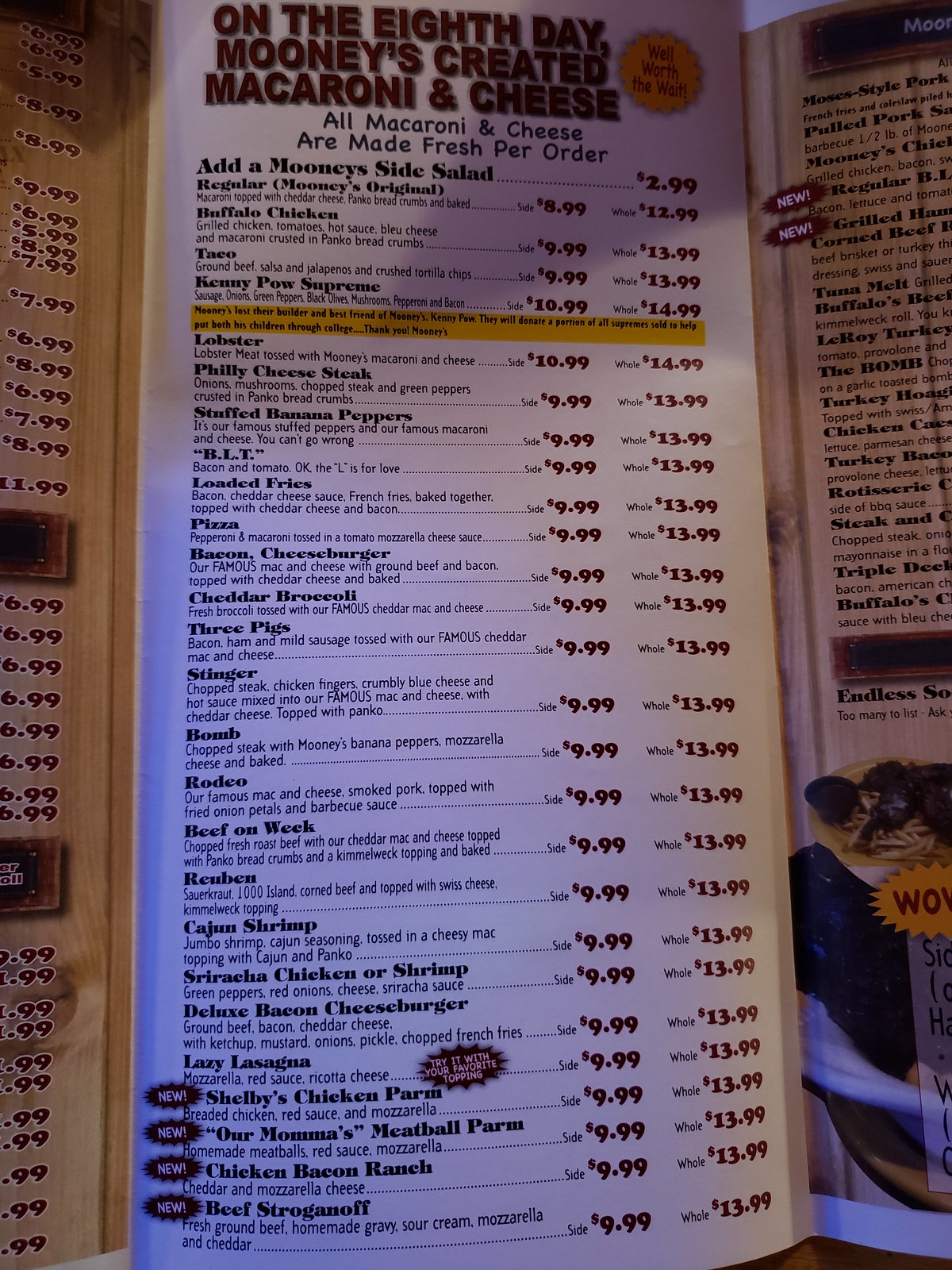This photograph captures a detailed view of a restaurant menu displayed against a white background. The menu is encased in a black border with the playful phrase, "On the 8th day, Mooney's created macaroni and cheese," written in red letters. The menu offers a variety of macaroni and cheese dishes, all made fresh per order.

Highlighted with black text, it states that customers can add a Mooney's side salad for $2.99. The prices for the dishes are categorized based on portion size: a side portion typically priced at $9.99 and a meal portion at $13.99.

Here is a meticulous list of the available dishes and their respective prices:
- **Mooney's Original**: $8.99 (side), $11.99 (meal)
- **Buffalo Chicken**: $9.99 (side), $13.99 (meal)
- **Taco**: $9.99 (side), $13.99 (meal)
- **Kenny Power Supreme**: $10.99 (side), $14.99 (meal)
- **Lobster**: $10.99 (side), $14.99 (meal)
- **Philly Cheesesteak**: $9.99 (side), $13.99 (meal)
- **Stuffed Banana Pepper**: $9.99 (side), $13.99 (meal)
- **BLT (Bacon and Tomato)**: $9.99 (side), $13.99 (meal)
- **Loaded Fries**: $9.99 (side), $13.99 (meal)
- **Pizza**: $9.99 (side), $13.99 (meal)
- **Bacon Cheeseburger**: $9.99 (side), $13.99 (meal)
- **Cheddar Broccoli**: $9.99 (side), $13.99 (meal)
- **Three Pigs**: $9.99 (side), $13.99 (meal)
- **Slinger**: $9.99 (side), $13.99 (meal)
- **Rodeo**: $9.99 (side), $13.99 (meal)
- **Beef on Weck**: $9.99 (side), $13.99 (meal)
- **Reuben**: $9.99 (side), $13.99 (meal)
- **Cajun Shrimp**: $9.99 (side), $13.99 (meal)
- **Sriracha Chicken or Shrimp**: $9.99 (side), $13.99 (meal)
- **Deluxe Bacon Cheeseburger**: $9.99 (side), $13.99 (meal)
- **Lazy Lasagna**: $9.99 (side), $13.99 (meal)
- **Shelby Chicken Parm**: $9.99 (side), $13.99 (meal)
- **Our Mama's Meatball Parm**: $9.99 (side), $13.99 (meal)
- **Chicken Bacon Ranch**: $9.99 (side), $13.99 (meal)
- **Beef Stroganoff**: $9.99 (side), $13.99 (meal)

The menu’s elegant design and comprehensive listing make it easy for diners to explore their delicious macaroni and cheese options.